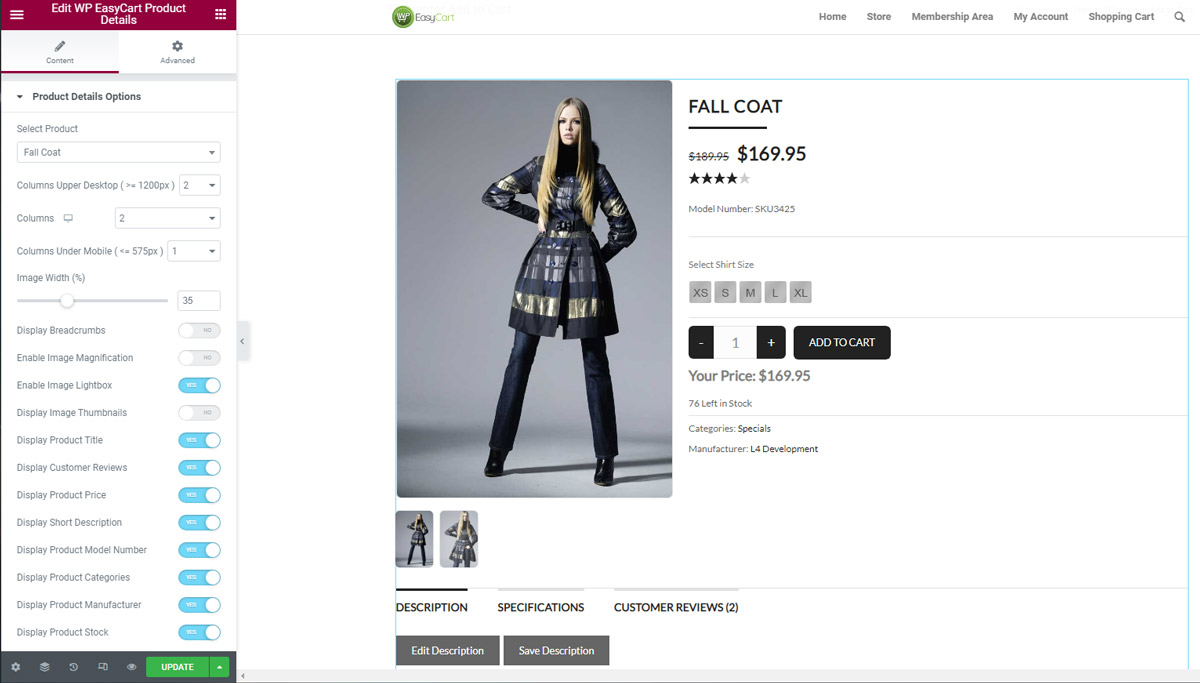A detailed image caption: 

The image features a woman dressed in a stylish fall outfit against a white background. She is wearing a jacket, pants, and boots. The fall coat is priced at $169.95 (previously $189.95). It has received a rating of four stars. The model number of the coat is SKU3425.

There are options for selecting skirt sizes, which include XS, S, M, L, and XL. Additionally, there is a quantity selector with a "1" in the middle and a minus sign to the left and a plus sign to the right. A gray rectangle displays the prompt "Add to Cart" in white text. 

The coat is currently priced at $169.95, and there are 76 units left in stock. The item falls under the category "Specials" and is manufactured by L for Development. 

Additional details include sections for "Subscription," "Specifications," and "Customer Reviews," with the latter showing a count of two reviews. There are also two gray rectangles labeled "Edit Description" and "Save Description."

At the top of the image, there are navigation options labeled "Home," "Store," "Membership Area," "My Account," and "Shopping Cart," as well as a magnifying glass icon denoting the search function.